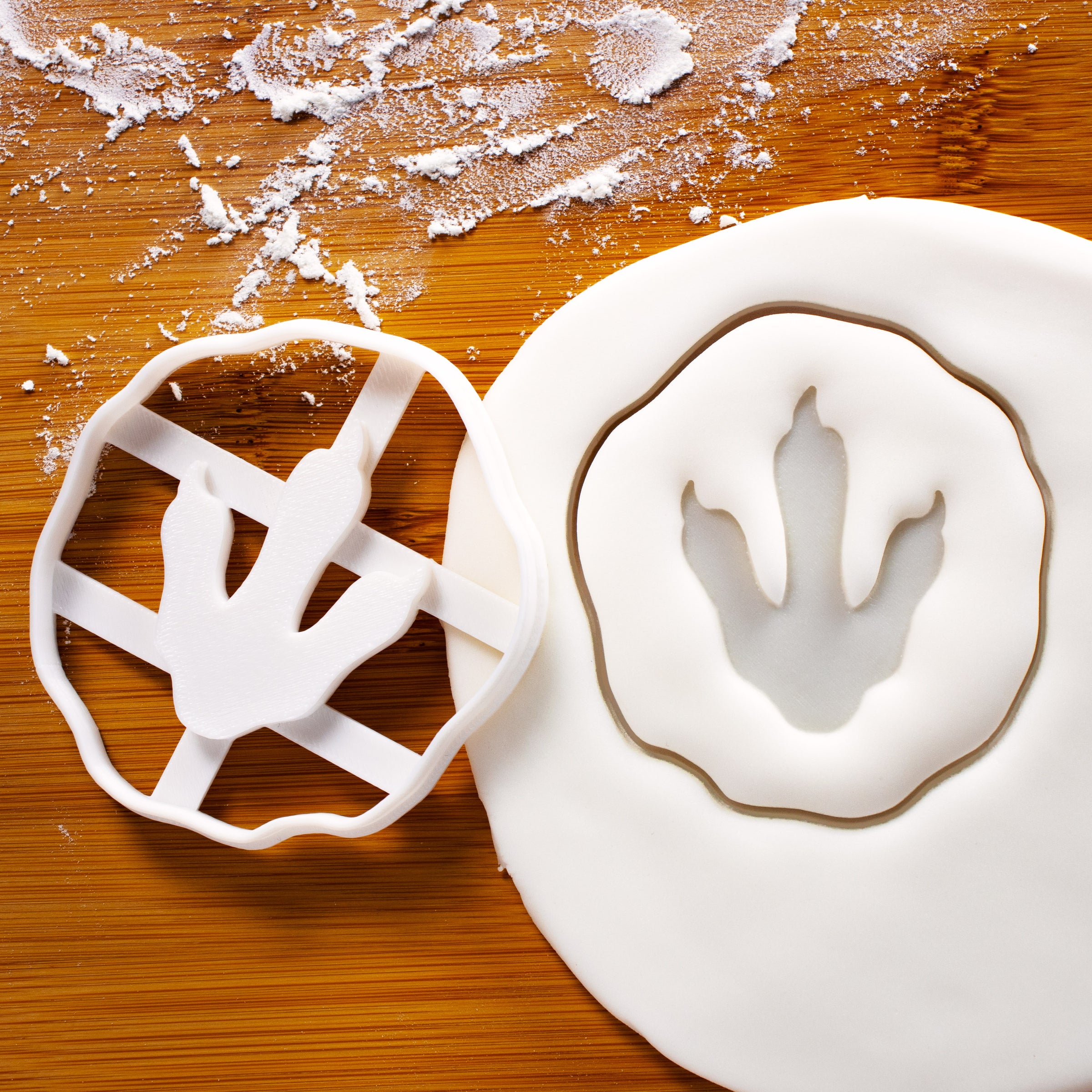The image depicts a scene likely computer-generated, set on a wooden table or cutting board, where someone appears to be baking cookies. The focus is on a clean, white circle of dough on the right side, which stands out against the messy, flour-strewn wooden surface, indicating that the baking process has been underway for some time. A distinctive white plastic cookie cutter lies upside down on the left side of the dough, peculiarly designed in the shape of a dinosaur or bird foot, showcasing three toes with claws. This cookie cutter has been pressed into the dough, leaving a clear footprint impression surrounded by an imperfect circle. This footprint mark indicates that it's ready to be separated from the rest of the dough for baking, eventually transforming into a cookie shaped like a dinosaur foot. The stark whiteness of the dough, almost resembling play dough, adds to the whimsical and possibly humorous nature of the scene.